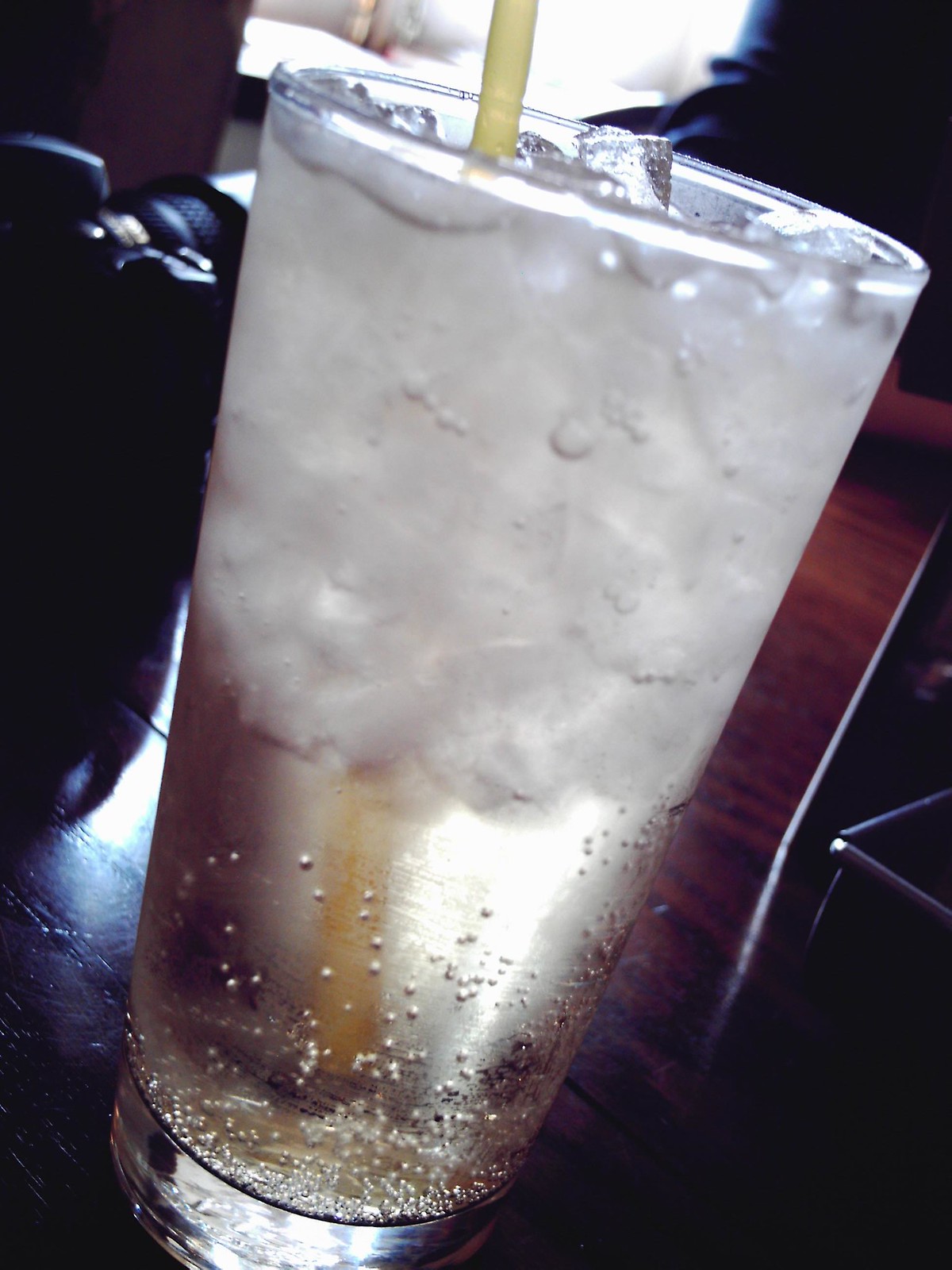In this color photo, the focal point is a tall, crystal-clear drinking glass filled with a transparent, bubbly liquid, likely a carbonated soft drink such as Sprite or 7-Up. The glass is diagonally tilted toward the right-hand side of the image and is more than half-filled with cubed ice. A thin, light yellow plastic straw emerges from the left side of the glass, extending beyond the top edge of the image. The beverage within the glass is effervescent, with numerous bubbles clustered at the bottom and rising along the sides. The background features a dark brown, almost mahogany wooden surface. To the left of the glass, there appears to be a dark table with a chair pulled away from it. The scene is dimly lit, though a bright, somewhat blurry white area near the top center suggests light coming through a window. The overall setting exudes a cozy, intimate atmosphere, accentuated by the play of light and dark shadows.